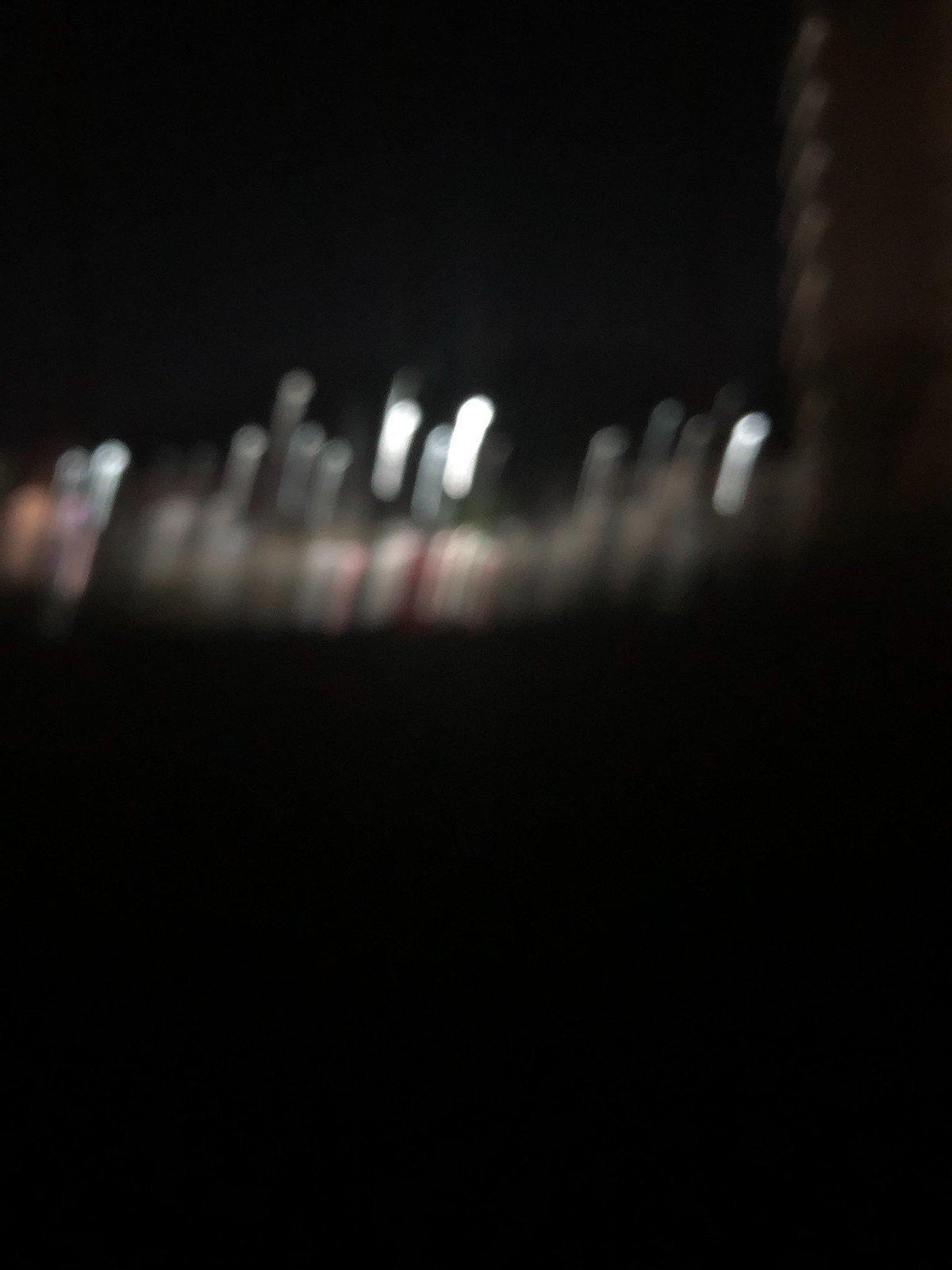This is an extremely blurry nighttime photograph predominantly engulfed in darkness. In the upper middle to upper right section, there is a cluster of lights displaying various colors, including white, orange, yellow, red, pink, black, and brown. However, due to the blurriness, it's difficult to make out specific objects or details, and the image is highly indeterminate. Amongst these blurred lights, there appears to be two twisted wires, possibly leading to a structure wrapped around a post, although this too is indistinct. The rest of the picture remains pitch black with no discernable objects, text, or subtitles, making it nearly impossible to identify any distinct features.